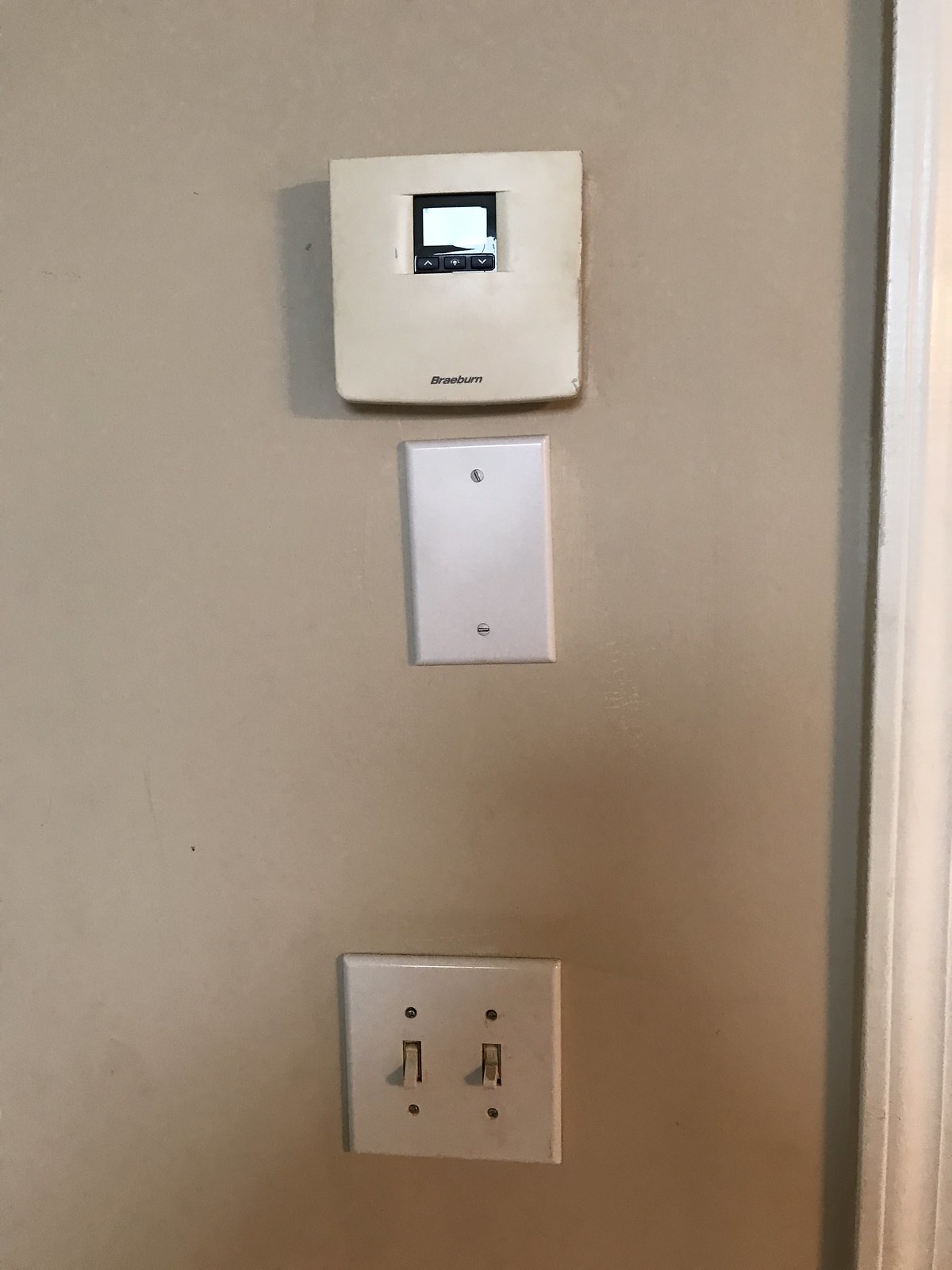The image showcases a beige-pink wall with white trim visible on the right side. Attached to the wall are three panels arranged vertically. At the bottom, there is a double light switch panel with a white cover and four screws, two positioned under each switch. The switches, which are in an off-white hue and slightly marked with paint splotches, both point downward. Just above, there is a slightly tilted white blank panel, also screwed to the wall. At the top of the arrangement, there is a rectangular off-white thermostat from the brand Braeburn, indicated by smaller lettering at the bottom. The thermostat features an inset screen with an up arrow, a down arrow, and a plus sign, though the screen itself appears damaged with a black splotch marring its digital green display.